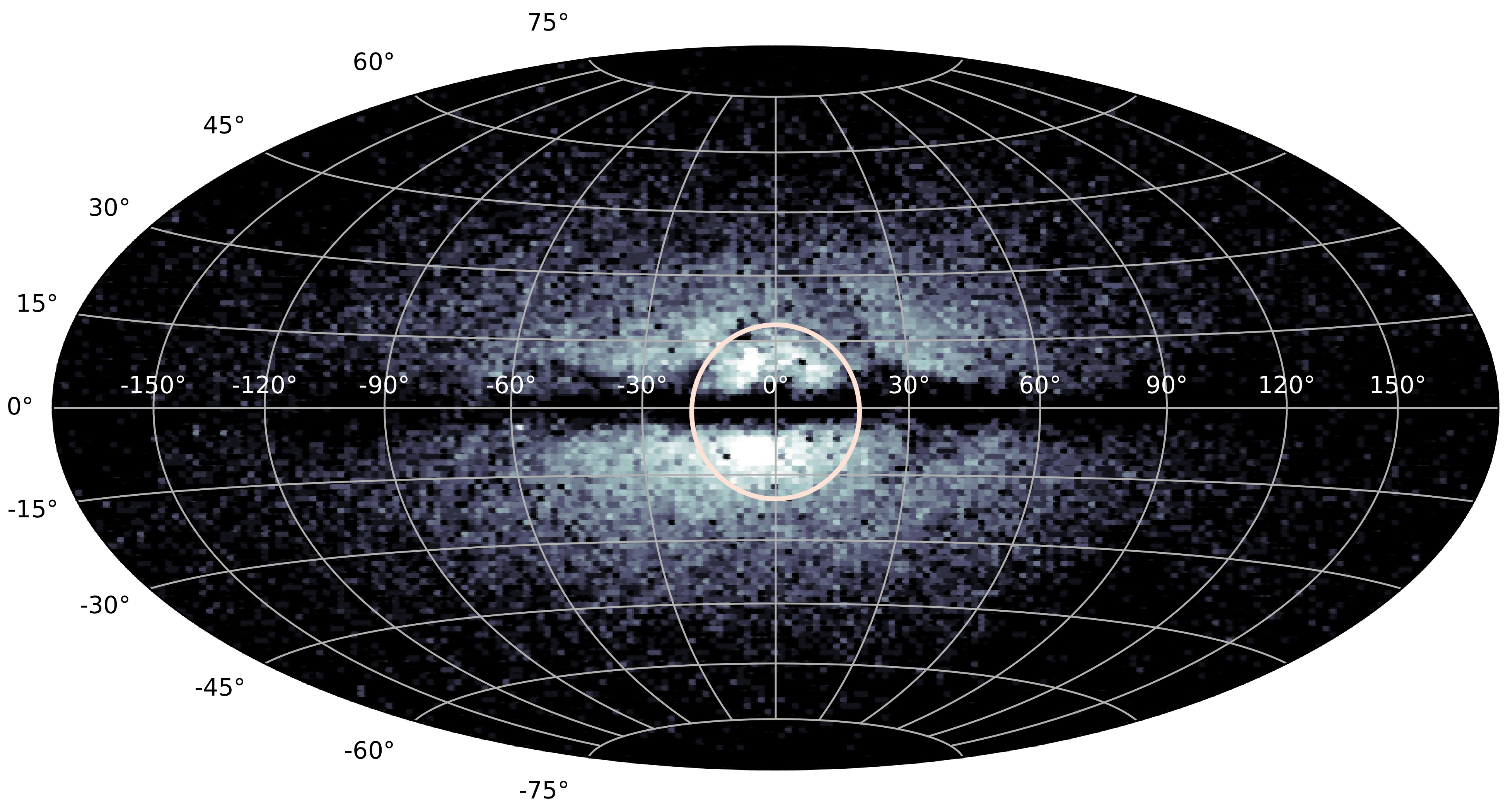This black and white image presents an astronomical feature situated against a black background, depicted within an elongated oval shape that stretches left to right. At the center of this oval, a pixelated representation appears, likely indicative of clustered stars or celestial bodies, creating a pattern of varying brightness—darker on the outskirts and lighter at the center. Overlaid on this image is a symmetrical grid composed of curved latitude and longitude lines, denoted in white. These lines include a straight horizontal axis through the center, marked at zero degrees. This horizontal axis extends from -150 to +150 degrees, while the vertical axis ranges from -75 to +75 degrees, with degrees labeled on the left-hand side. The center of the image features a prominent white circle at the zero-degree mark, highlighting the midpoint of this celestial mapping. The blending of scientific grid lines with the pixelated depiction of space creates an intricate and detailed astronomical visualization.